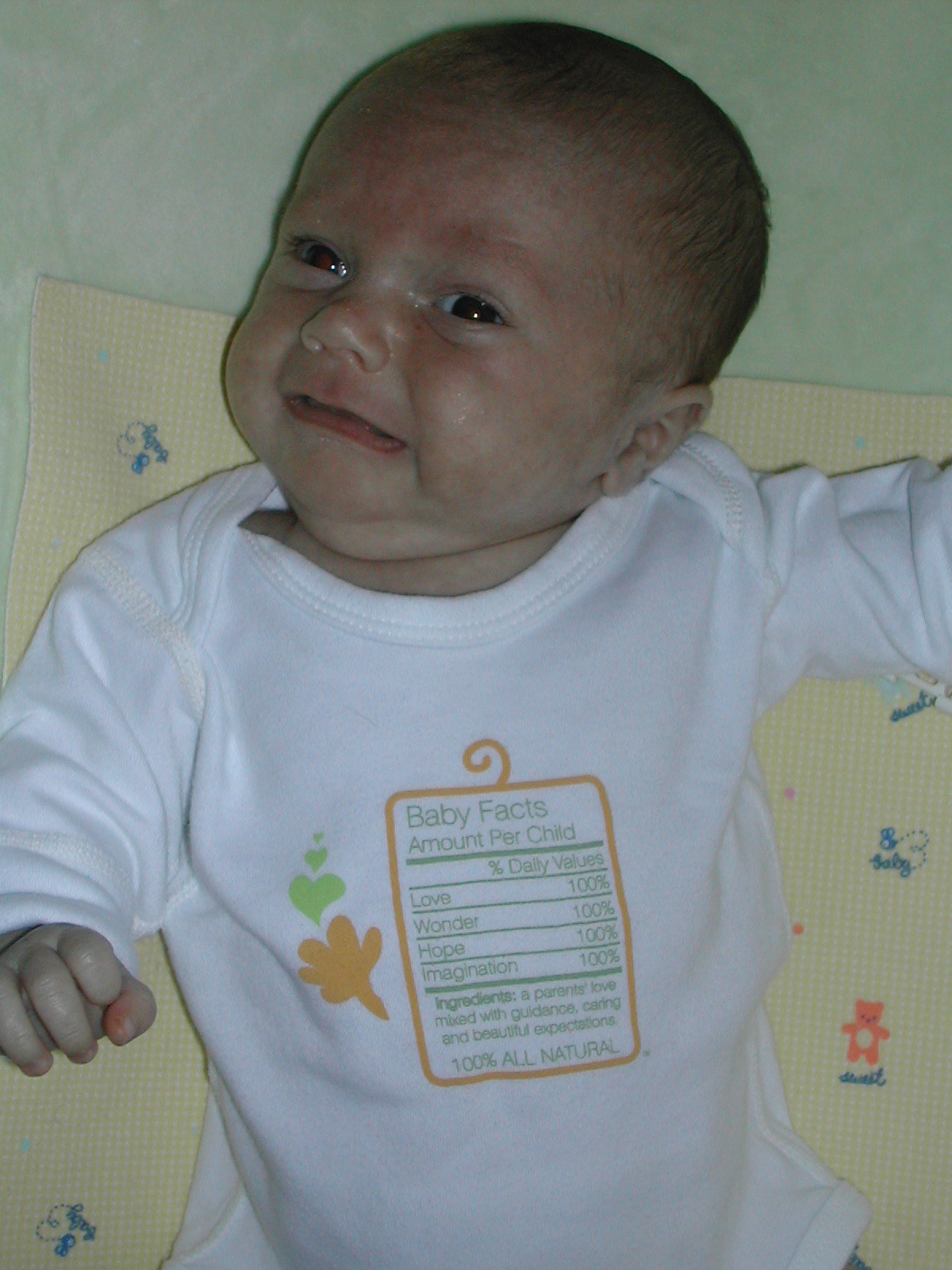The image depicts a Caucasian baby, likely less than a year old, lying on a soft yellow blanket adorned with teddy bears and bumblebees. The baby, with short brown hair, is wearing a white onesie decorated with small green hearts and a tiny orange leaf. The onesie features a graphic resembling a nutritional label, labeled "Baby Facts." The text includes "Amount per child," "Percentage daily values," followed by "Love 100%," "Wonder 100%," "Hope 100%," and "Imagination 100%." It further lists the "Ingredients" as "A parent's love mixed with guidance, caring, and beautiful expectations," concluding with "100% all-natural." The baby appears to be on the verge of crying, adding an emotional touch to this endearing scene.